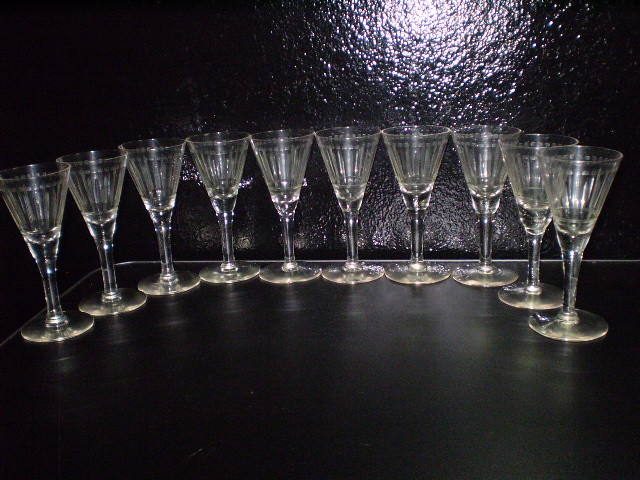The image captures a stylish arrangement of ten transparent champagne flutes with vertical etchings, meticulously organized in a semicircle on a sleek black tabletop. The backdrop features a textured black wall, against which the light from the camera's flash reflects, adding a subtle glow to the scene. The delicate patterns on the glasses and their reflective bottoms enhance the elegance of this bar or club setting.